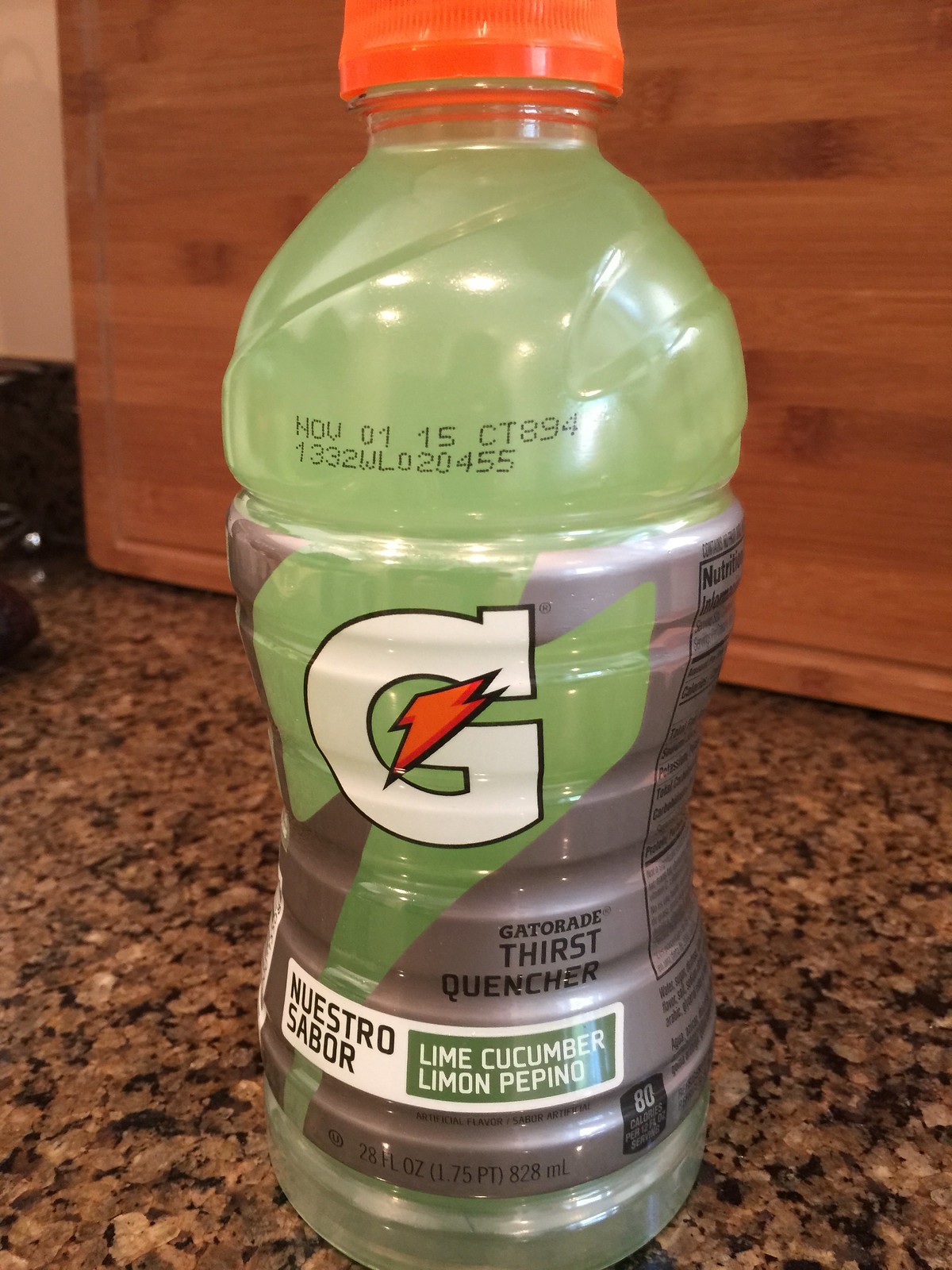The photograph, taken indoors within a kitchen setting, prominently features a bottle of Gatorade. The scene is set against a backdrop that includes a wooden or bamboo cutting board standing upright, and a brown, stone-like countertop. The Gatorade bottle is made of clear plastic, showcasing its pale green liquid content. It is topped with an orange screw-off cap. The label on the bottle displays a distinct white "G" accompanied by an orange lightning bolt, and it reads "Gatorade Thirst Quencher Lime Cucumber." Additionally, the bottle is stamped with the date November 01 and the code 15 CT 894.